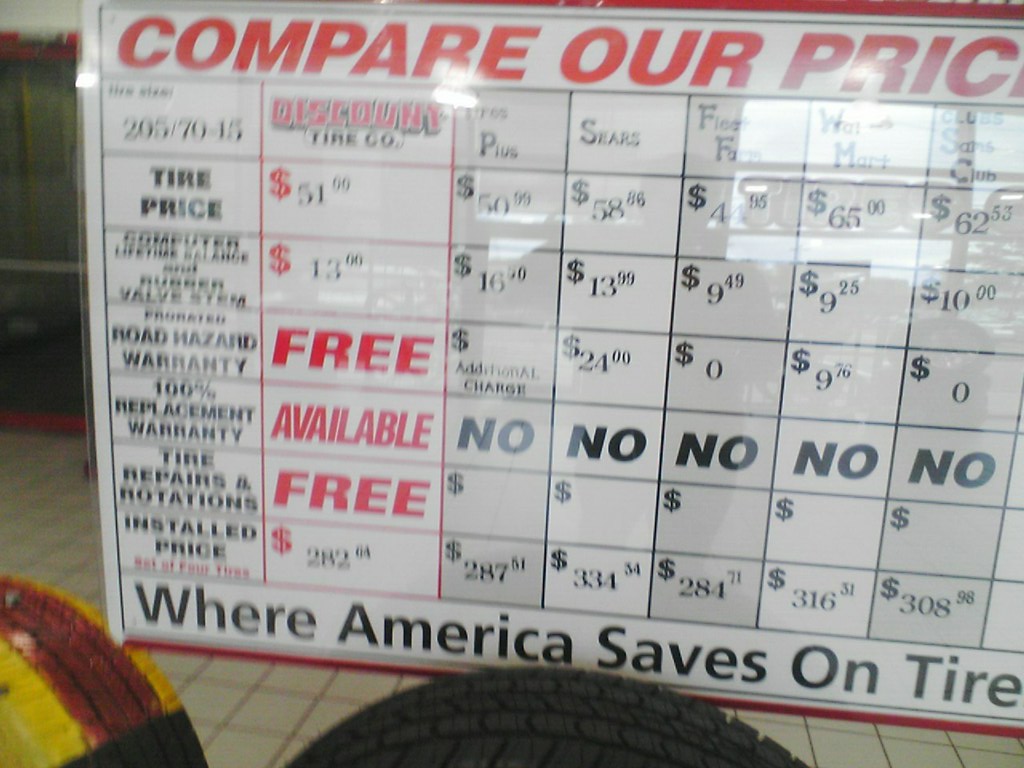In this photograph of a pricing chart at an auto repair place, the prominent feature is a large white sign with a black grid layout, resembling a calendar. At the top of the sign, in red text, it says "Compare Our Prices," below which the chart lists various tire-related services and their prices. 

The first column showcases "Discount Tire Company" with the tire size specified as 205/70-15. Following this, the chart details the costs for different aspects such as "Tire Price" ($51), "Computer Lifetime Balance & Rubber Valve Stem" ($13), "Prorated Road Hazard Warranty" (Available), "100% Replacement Warranty" (Free), "Tire Repairs and Rotations" (Free), and "Installed Price" (AB264). 

Other companies listed for comparison include Tires Plus, Sears, Fleet Farm, Walmart, and Sam's Club, with their respective prices shown in the columns. The final row illustrates the installed prices: Tires Plus ($287.51), Sears ($334.34), Fleet Farm ($284.71), Walmart ($316.31), and Sam's Club ($308.98), highlighting Discount Tire Company's competitive or lower rates for some services.

The background includes beige-tiled flooring, and two tires, one of which is painted yellow with a red stripe. The bottom of the sign reads "Where America Saves on Tires," encapsulating the price comparison message. However, the image is somewhat obscured by reflections and light, making some details difficult to discern.